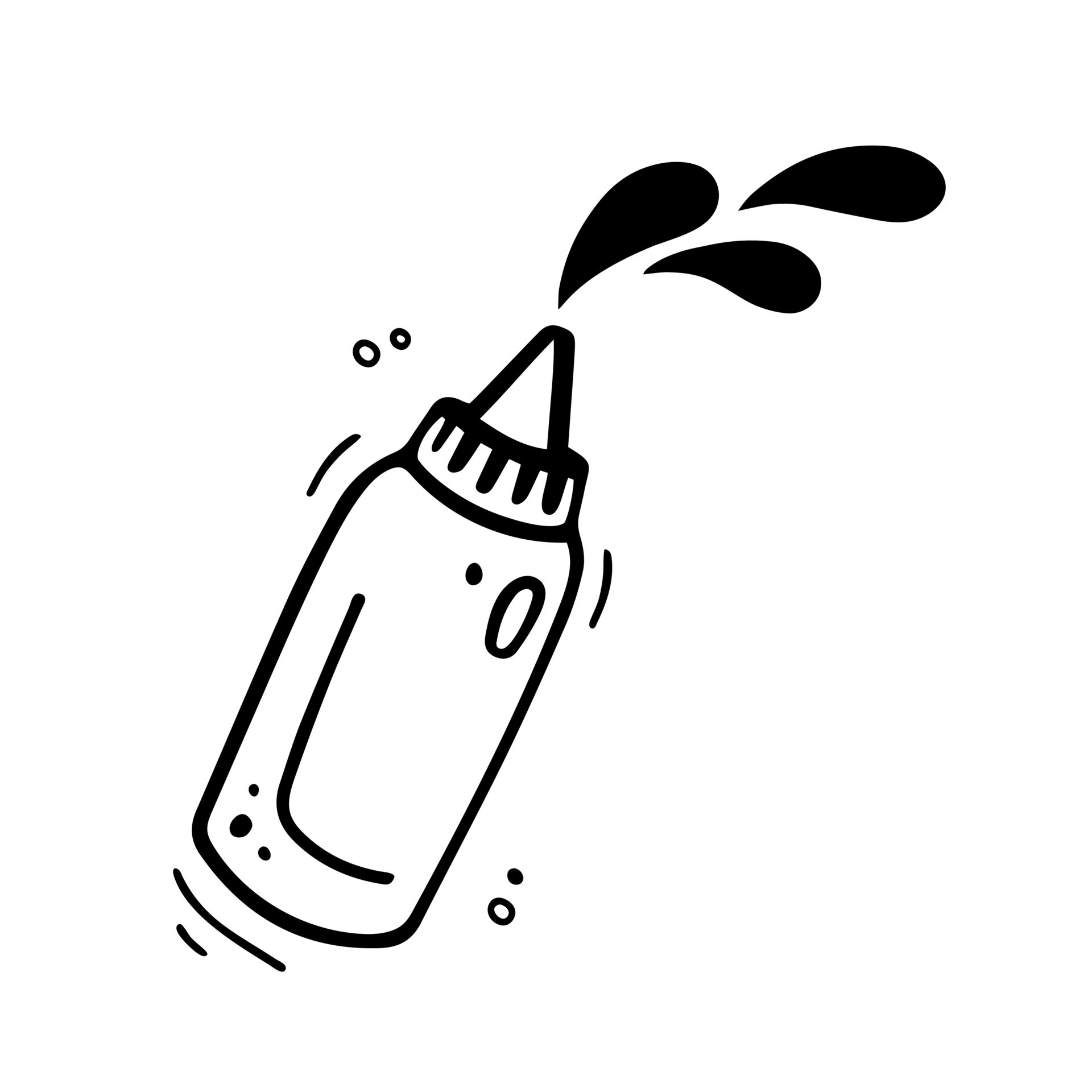This image is a detailed black and white drawing, likely digital art, depicting a bottle, which could be either a ketchup or baby bottle, outlined in black against a pure white background. The bottle, sloped positively from the bottom left corner upwards, appears to be shaken as indicated by animation markings around it. Its base is near the bottom left-hand corner, and it has a screw top with a perforated round shape and a triangular, beak-like nozzle. Emerging from this nozzle are three large black droplets, depicted just above it. Inside the bottle, a black 'L' shape enhances the impression of curvature. Additionally, there are small black dots near the bottom left corner, potentially representing bubbles, and other circles outlined in black. The overall illustration is reminiscent of clip art, often seen on websites, and emphasizes the motion of the liquid being squirted out.